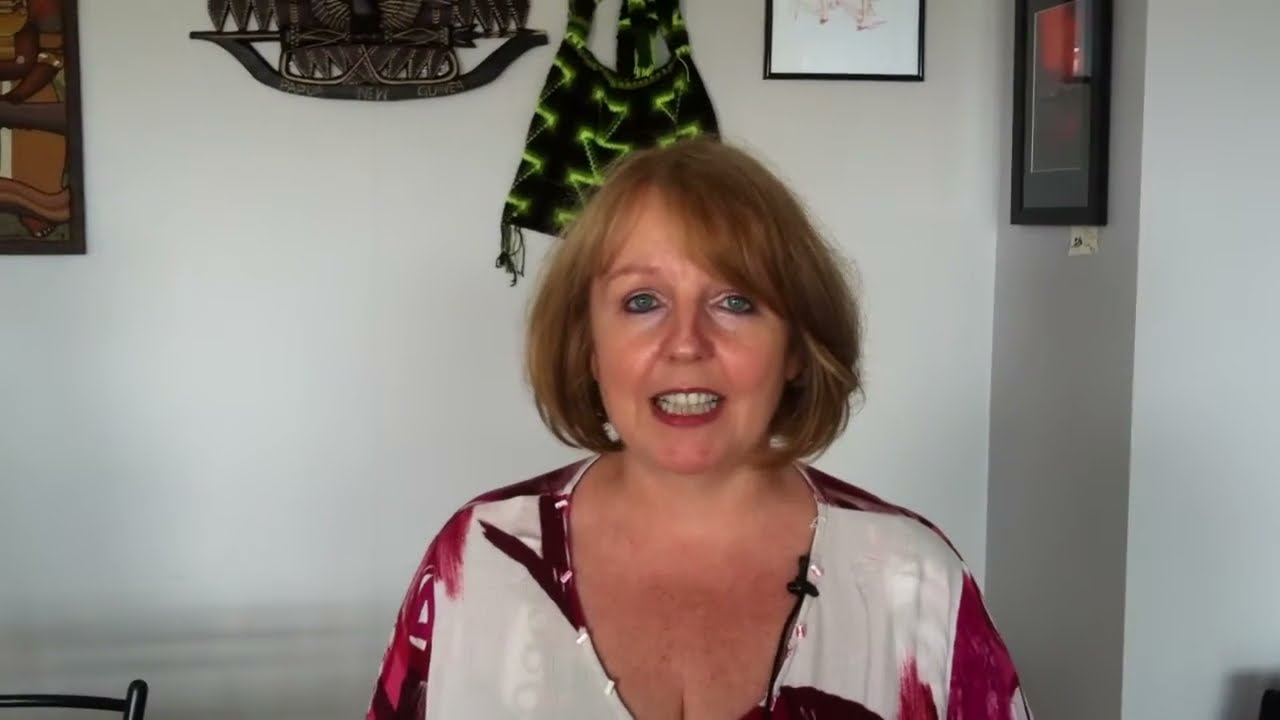The photograph, taken indoors, features a woman standing at the center, captured from the chest level up. She appears to be in her late 40s or early 50s, with strawberry blonde, chin-length hair that frames her face. Her striking blue-green eyes stand out, and she is smiling, displaying her teeth with a touch of red lipstick. She is wearing a very low-cut blouse with a gauzy texture and abstract stripes of maroon, black, and white, revealing the top of her cleavage. The background reveals a light gray or off-white wall adorned with various items, including art and photographs. Notable background elements include a black bag with neon green triangles hanging behind her head, a framed abstract picture on the upper left, and several other framed artworks along with metal wall decor. A menorah plaque is visible, and to the lower left, the top of a chair peeks into the frame. The image exudes a professional yet artistic atmosphere, suggesting it might be used for promotional purposes, potentially in real estate or similar fields.